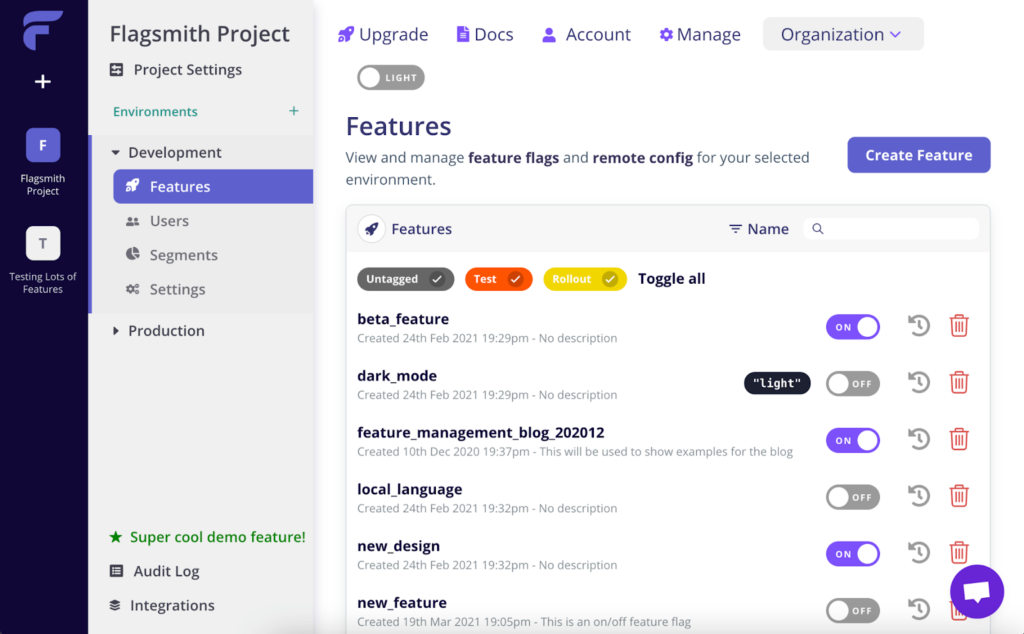This image is a screenshot of a webpage from the Flagsmith Project, displayed on a computer screen. The interface is divided into several distinct areas, each serving a specific function. On the left side of the screen, there is a dark blue vertical banner, likely serving as a navigation pane. On the right side, a series of tabs is displayed against a white background, providing access to various sections of the Flagsmith Project.

In the central portion of the screen, there is a grayish banner with black lettering, which appears to list different features available within the Flagsmith Project. Below this banner, multiple selections can be seen, each accompanied by toggles that allow users to enable or disable specific features. The overall interface seems to be focused on configuring and managing the features and settings of the Flagsmith Project.